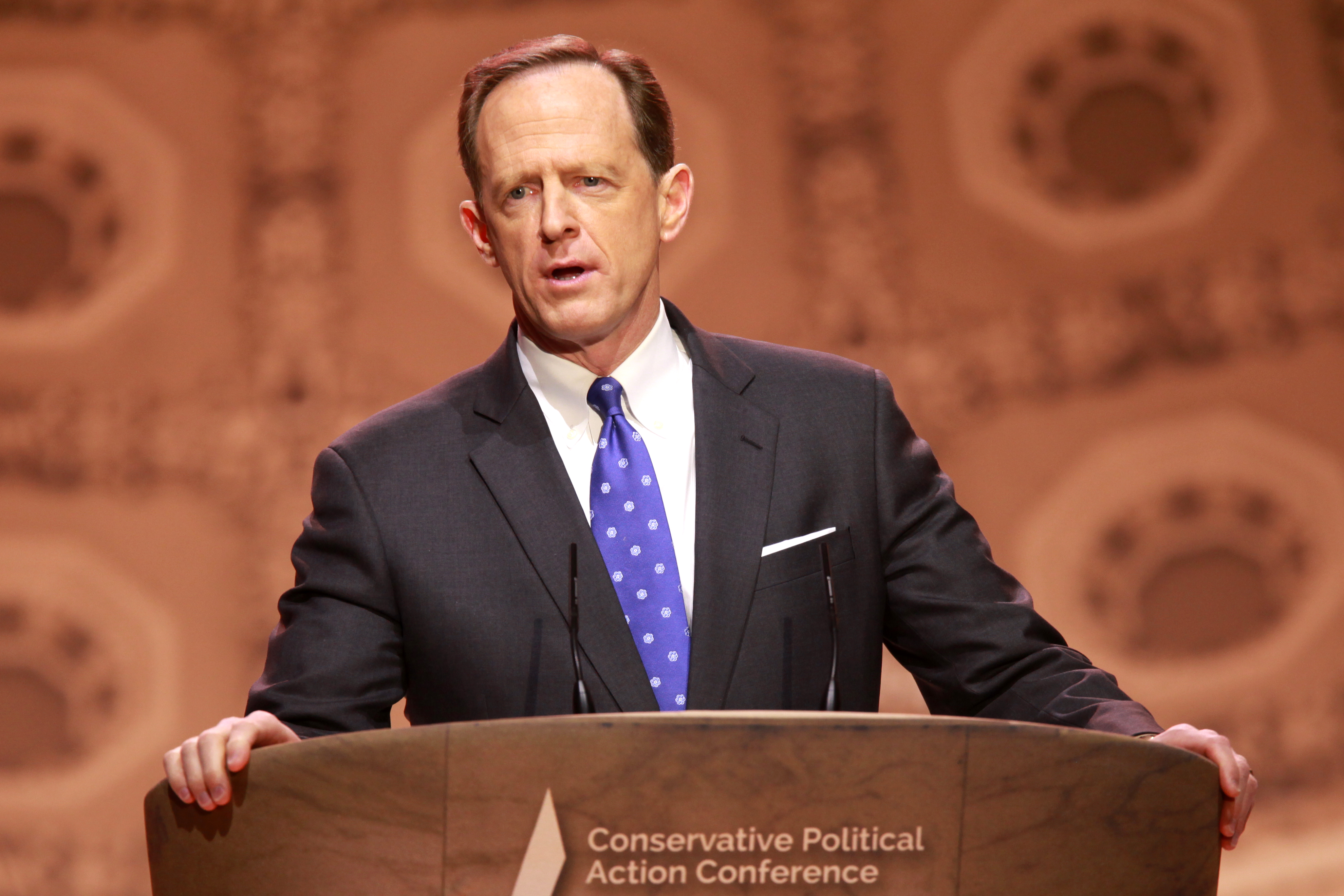A man stands behind a rounded, brown wooden podium with his hands gripping the edges in a firm, assertive stance. He wears a dark-colored suit, either black or dark gray, paired with a white shirt and a blue tie adorned with white dots. A white handkerchief neatly peeks out from one of his suit pockets. His hair is brown and slightly receded, revealing a pronounced forehead, and he has notable ears. He has a serious expression with his mouth slightly open, as if addressing an audience. Two skinny microphone wires extend from the podium. The front of the podium features beige letters spelling out "Conservative Political Action Conference" alongside a diamond-shaped emblem. The background is blurred with a mix of beige and brown colors, featuring indistinct circular designs, creating the impression of a formal political event setting.